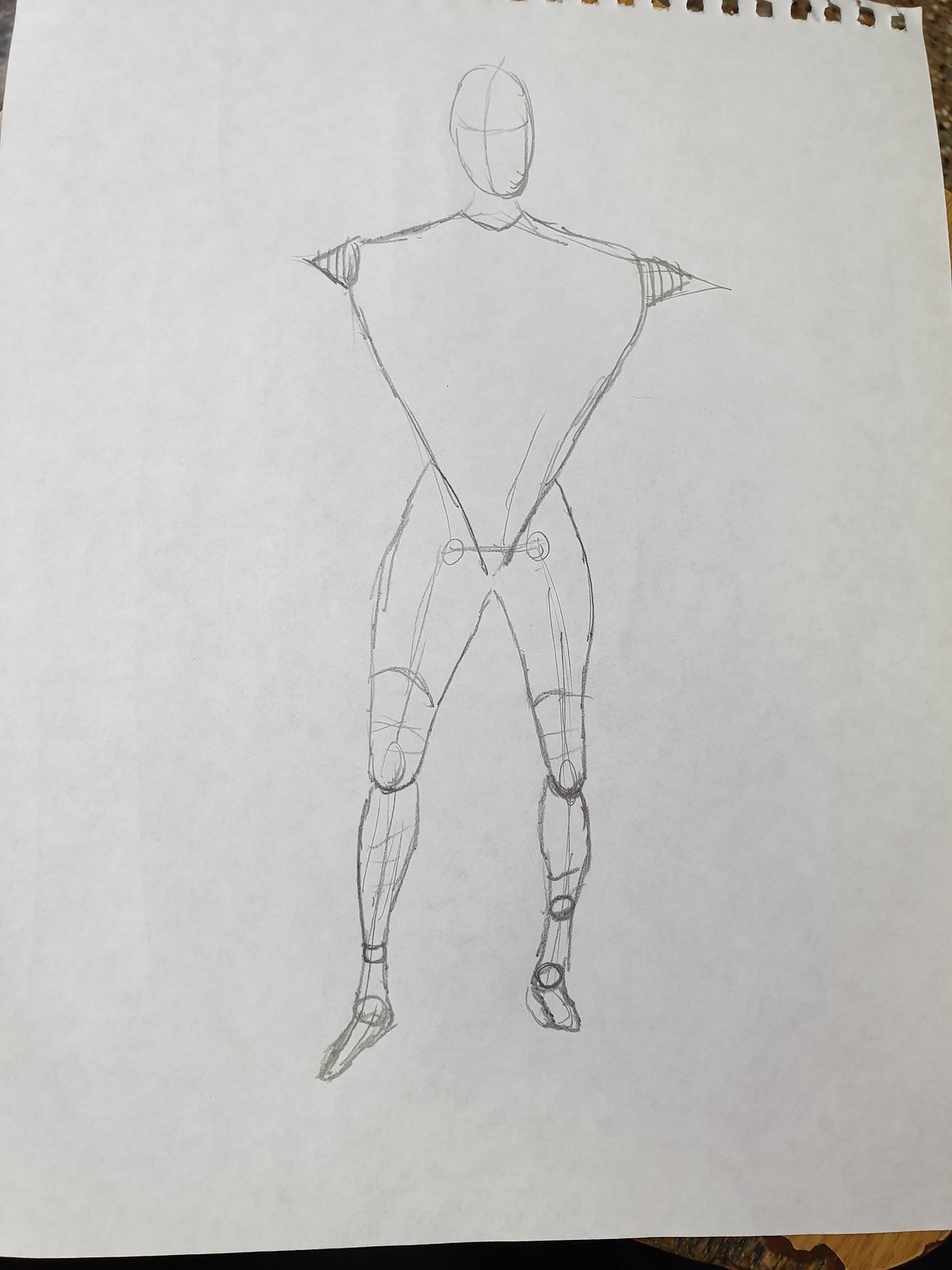This image shows a pencil sketch on a piece of paper torn from a spiral-bound sketchbook, evident from the hole punches visible at the top edge. The paper, resembling thin, white printer paper, might be around A4 size. The photograph of the sketch also captures a hint of a darker surface beneath the paper, perhaps a wooden floor.

The drawing itself appears to be an amateur anatomical study, possibly created by a junior high or high school student. The human-like figure features an oval-shaped head with a cross of slightly curved lines indicating facial sections. The neck and broad shoulders transition into a distinct inverted triangular torso that tapers down to the crotch. Instead of arms, there are small triangular nubs extending from the shoulders. The legs show a basic framework with defined hips, thighs, knees, calves, ankles, and feet. Joints are indicated with circles at appropriate locations. While the sketch is simple and not highly detailed, it demonstrates a thoughtful approach to anatomical structure and proportion, suggesting potential for further development.